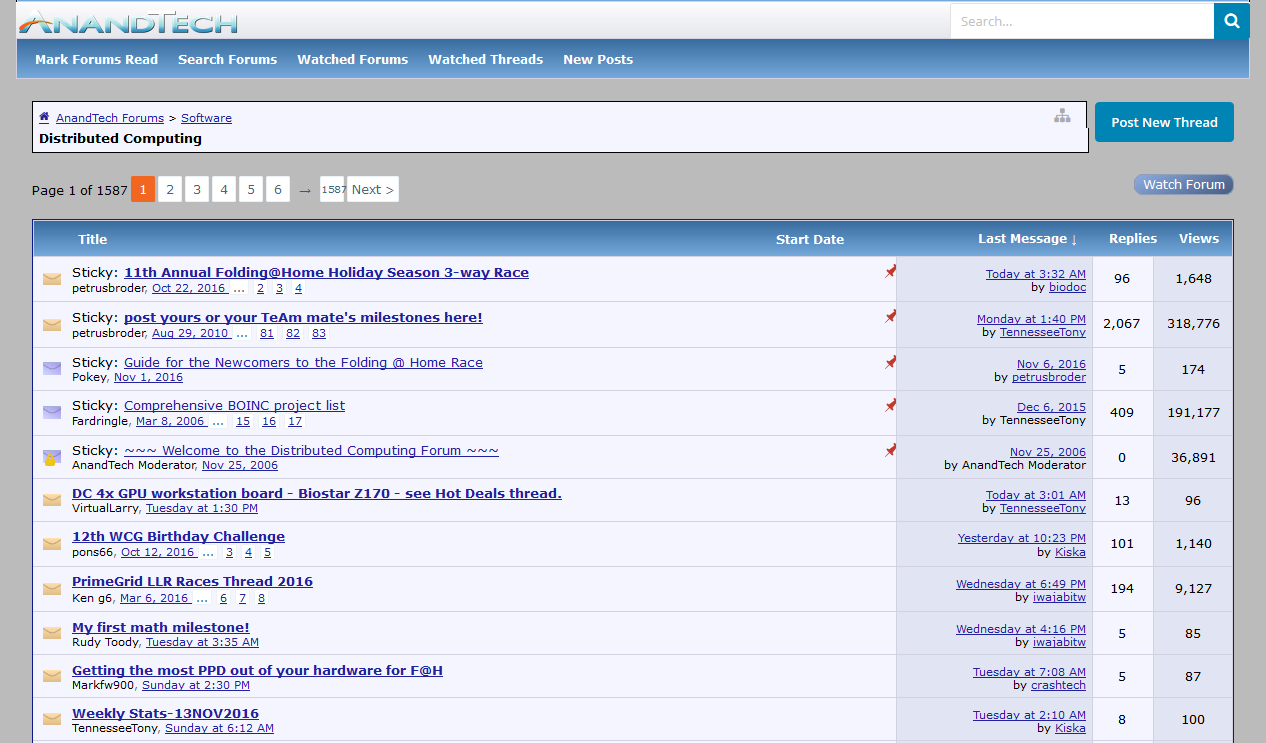This screenshot from a website showcases search results for files. The website has a grey background with a light grey header bar at the top. On the top left, there's a logo labeled "ANANDTECH," all in one word. On the top right, there's a search bar with a magnifying glass icon indicating the search functionality.

Below the header, there's a blue navigation bar with the following options: "Mark Forums Read," "Search Forums," "Watched Forums," "Watched Threads," and "New Posts." Beneath this navigation bar, a white result box displays the title "AnandTech Forums - Software - Distributed Computing" with a "Post New Thread" button in white on a dark teal background on the far right.

Below this result box, pagination information is shown: "Page 1 of 1587" on the left. Next to it, numbers from 1 to 6 are presented in white squares to navigate through pages, with page 1 highlighted in orange. Following the numbered squares are ellipses indicating more pages and the number "1587" representing the last page. A dark blue capsule-shaped "Next" button with a right arrow is on the far right.

On the same line, to the far right, there's a dark blue capsule-shaped button labeled "Watch Forum" in white. 

The results on page 1 are displayed in a table format beneath a header bar that transitions from dark blue at the top to a slightly lighter blue at the bottom. The columns are labeled as "Title," "Start Date," "Last Message," "Replies," and "Views." The table lists 11 results, each detailing the corresponding information under each column.